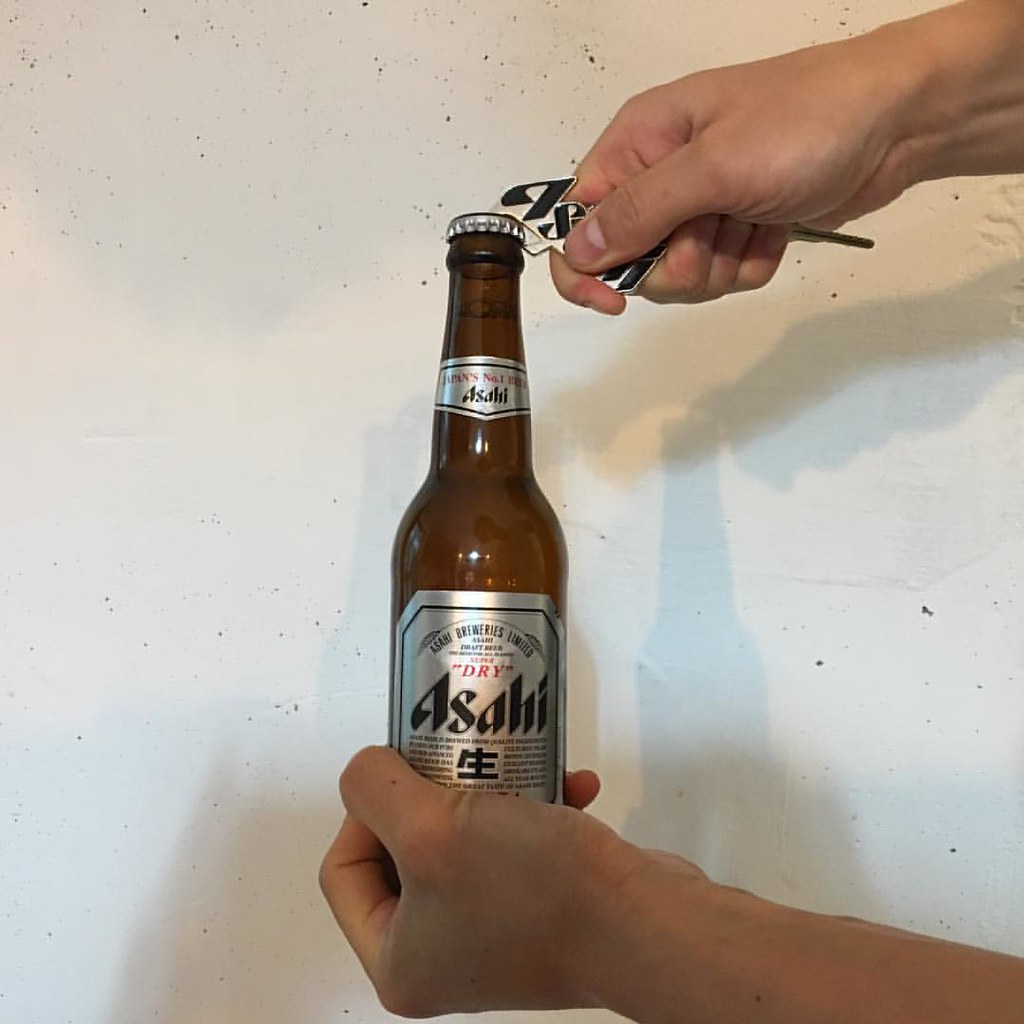In this detailed color photograph, we observe a close-up scene of someone opening a bottle of Asahi beer using an Asahi-branded bottle opener. The right hand, identifiable by the thumb facing towards the camera, is firmly gripping the bottle opener, which bears the brand's stylized black text, identical to the logo on the beer bottle's silver label. The left hand supports the brown glass bottle from the bottom. 

The bottle itself features a silver label with the brand name "Asahi" in bold black text, a smaller label around the neck which also displays the name in black text, and a silver metal cap. Additional text on the label includes "Asahi Breweries Limited" and "Dry," along with a round strip at the top stating "Japan’s number one beer," and what appears to be an Asian character in the middle.

The background of the image is a white surface speckled with random black spots, giving it a marble-like or dirty appearance. The shadows of the bottle and hands are prominently cast on this background, adding depth to the composition. The photo captures the moment just before the bottle cap is removed, highlighting the intricate details of the bottle and opener.